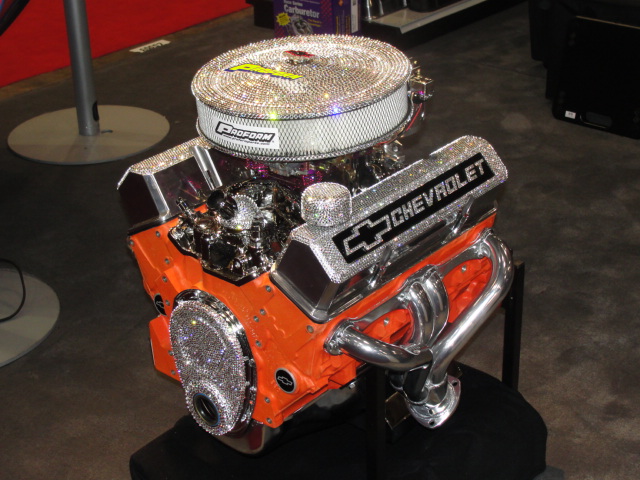The image showcases an elaborately decorated Chevrolet engine block, prominently positioned on a backdrop that resembles a black chalkboard-like floor—a surface which might actually be gray carpet with red accents noticeable in the upper left corner. Viewed from above and an angle, the engine sits within a black supporting frame. The engine block itself is vividly painted orange, with all the fixtures and fittings in shimmering, silver chrome, adorned with glittering, reflective stones for a blinged-out appearance. The middle of the engine features a radiant red section, further enhancing its vividness. The iconic Chevrolet logo and the word "Chevrolet" are clearly visible, outlined in black, on the side of the motor. Adding to its striking appearance, the air filter on top, which bears the label "Proform" in neon yellow letters, is similarly embellished with glittery decorations. The background features other indistinct objects and display stands that add context to this detailed and visually stunning photograph.